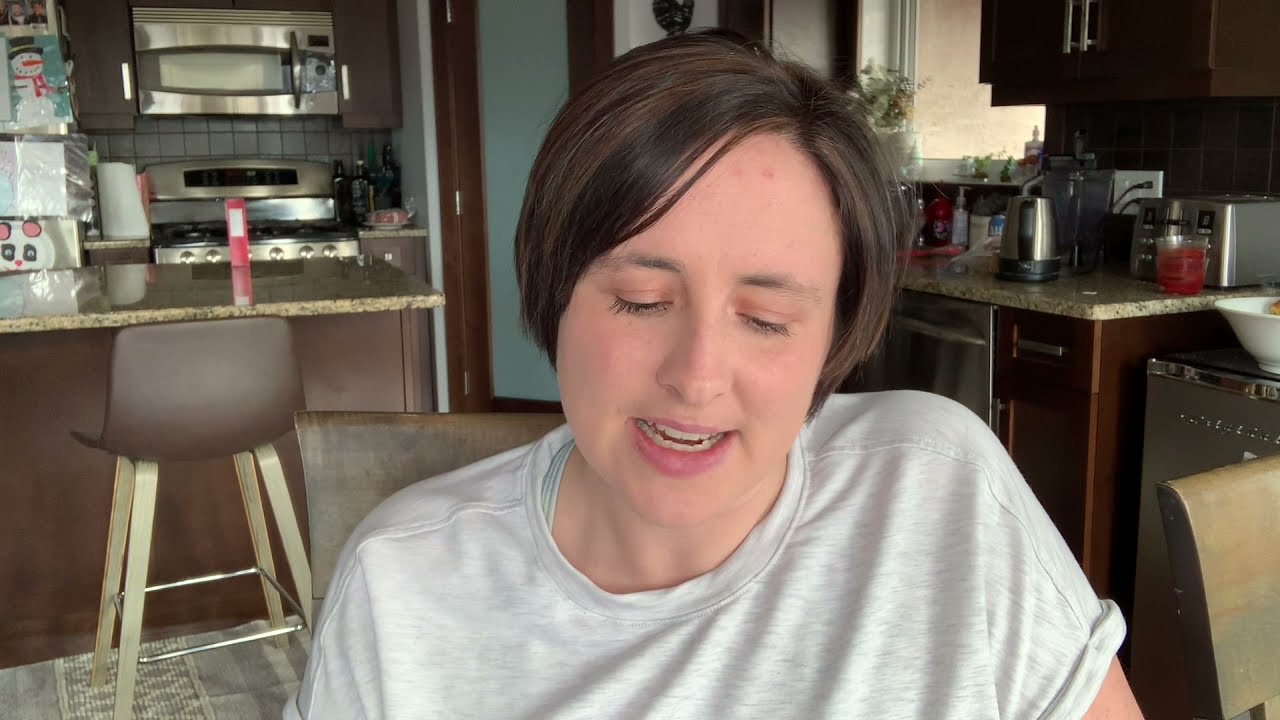In the image, a young woman, likely in her twenties, sits at the forefront of a modern kitchen, wearing a gray short-sleeved t-shirt and sporting a short bob haircut. She appears to be engaged in a conversation, possibly on her phone, as she looks downward with her mouth slightly open, revealing both her top and bottom teeth. The kitchen behind her features stainless steel appliances, including a stove, microwave, and possibly a mini-fridge. To the left side of the background, there is a refrigerator adorned with pictures, including one of a snowman. The kitchen also includes a brown marble-topped island with modern brown chairs, and to the right, various kitchen counters with small appliances like a coffee pot, toaster, and a white bowl on top of one counter. The counters are cluttered with bottles, paper towels, and food items. The woman’s complexion appears pale with a hint of redness as she focuses intently on her conversation.